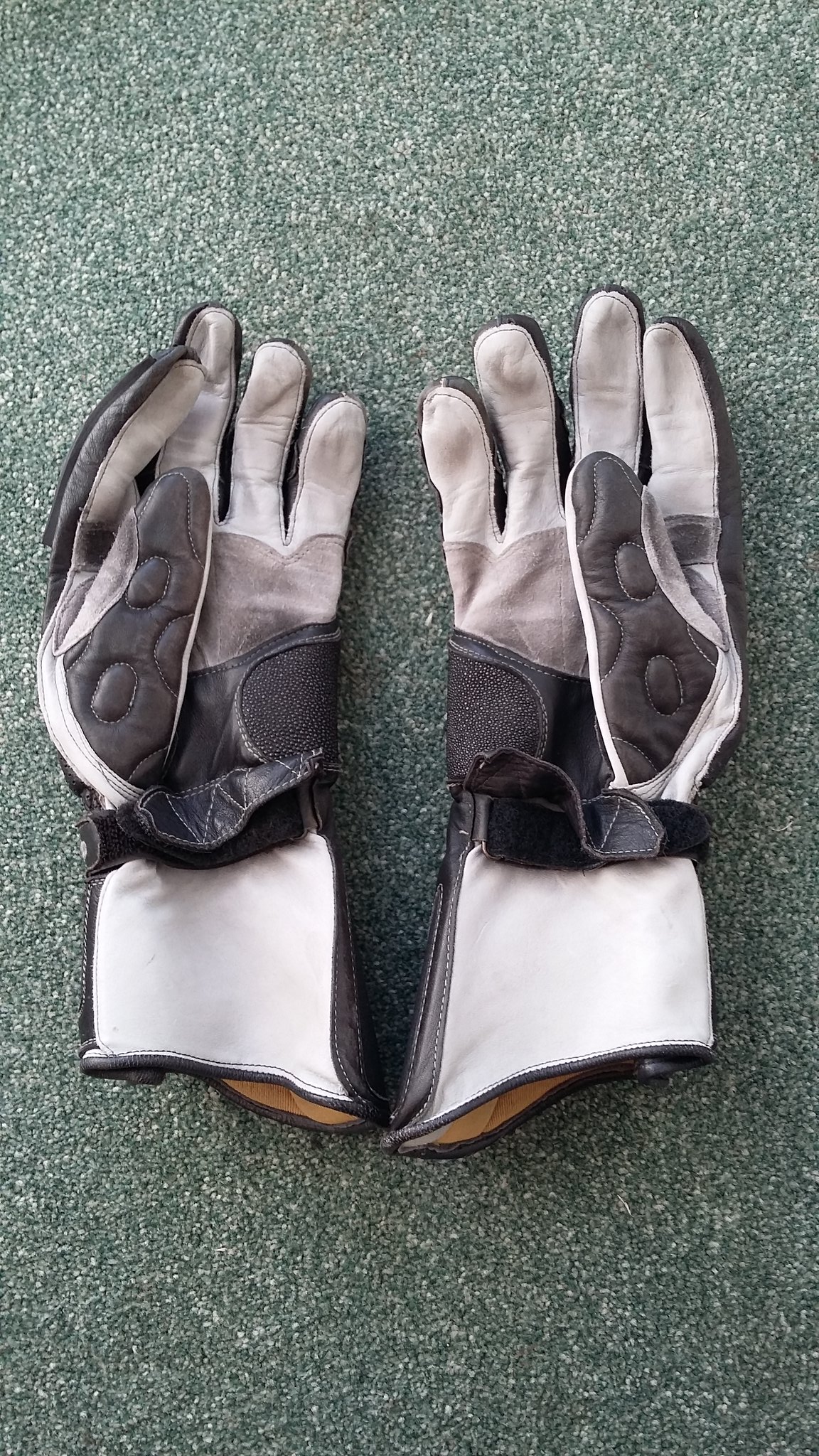The vertically rectangular photograph features a pair of gloves laid palm-side up against a textured green and white background, resembling either artificial turf or an off-green corkboard. The gloves appear primarily white on the fingers and cuffs, with distinguishing details such as a brown leather strip with Velcro running down the middle, a black strap around the wrist, and brown leather thumb areas embroidered with circular patterns. The thumbs are folded over the palms, revealing hints of an orange interior peeking out from the base. The left glove is positioned on the left side, and the right glove on the right, highlighting their symmetrical placement.